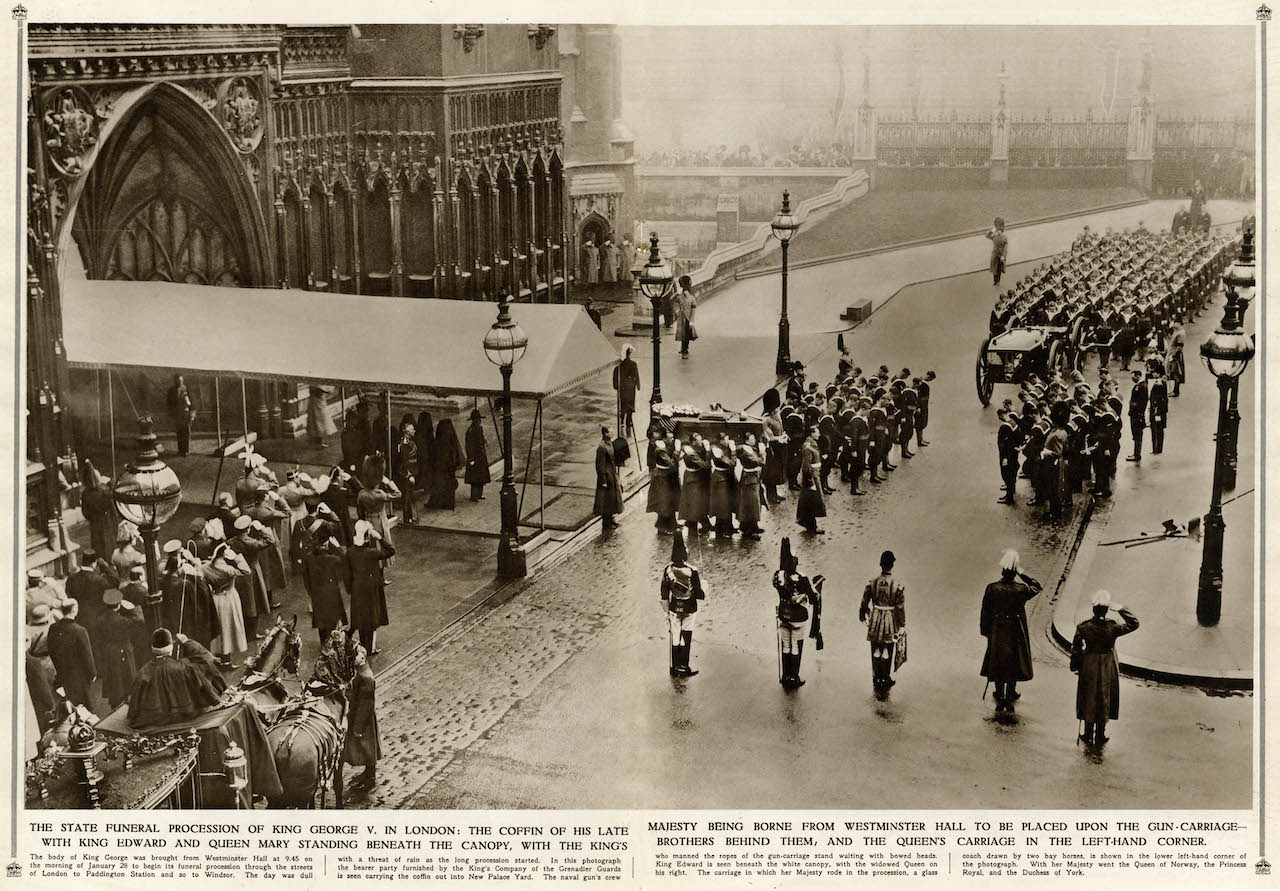The image is an antique black-and-white photograph, likely clipped from a newspaper, depicting the state funeral procession of King George V in London many years ago. The slightly yellowed paper, horizontal orientation, and black ink suggest it's an older, archived piece. Central to the scene is the late king's coffin being carried from Westminster Hall to the gun carriage. The procession is solemn and formal, with King Edward and Queen Mary standing beneath a canopy, the King's brothers positioned behind them, and the Queen's carriage visible in the left-hand corner. The event is attended by roughly 100-200 individuals, including military personnel, state officials, and possibly clergy, all saluting in respect. The atmosphere appears misty, in keeping with typical London weather, adding to the somber tone of the day. The crowd, comprising both officials and ordinary spectators, lines the street to pay homage, while the sounds of horses pulling carriages underscore the period setting.